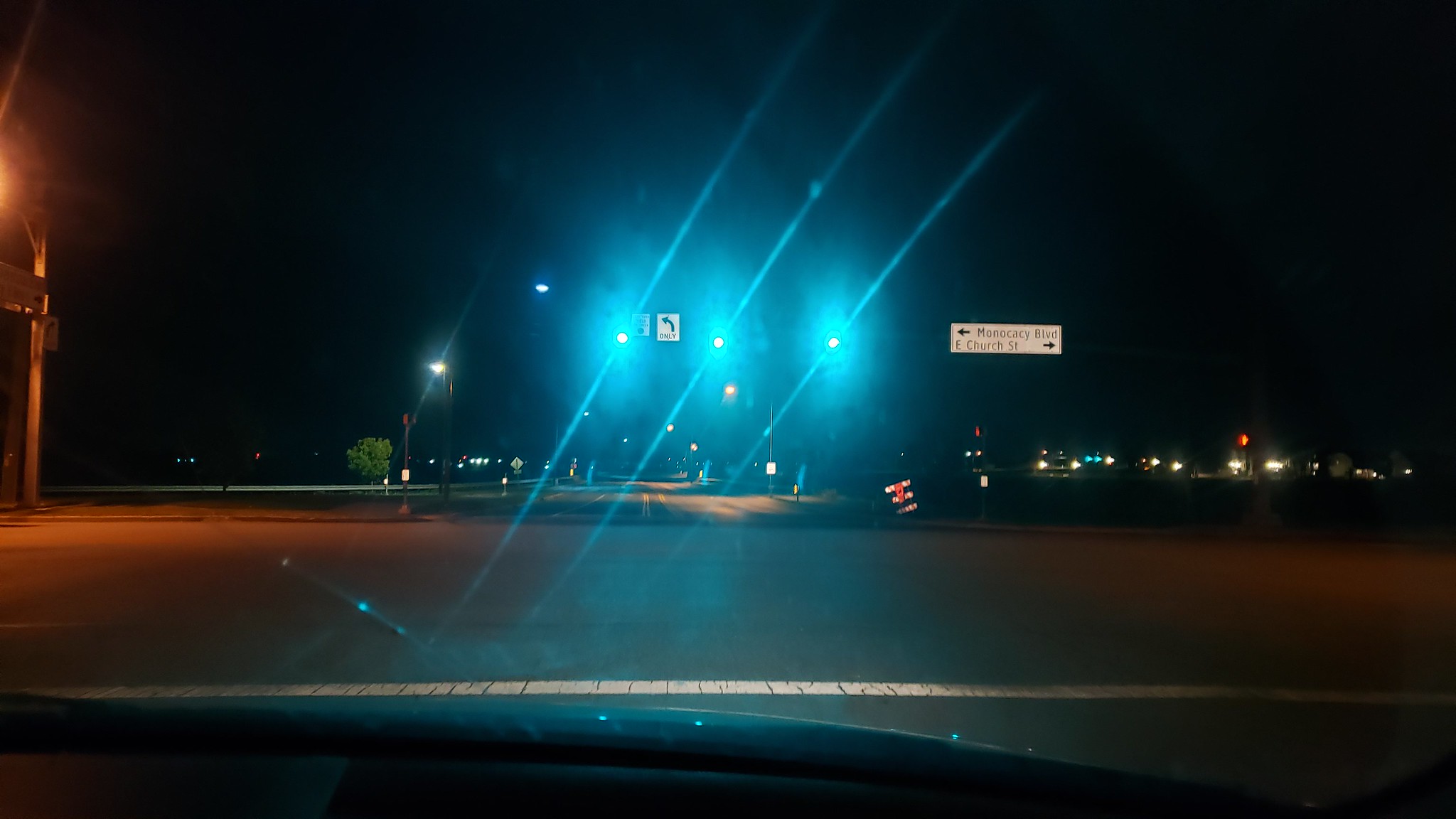A nighttime view from inside a car stopped at a traffic light, which has now turned green. The road ahead appears eerily empty, with no other vehicles in sight. The bright green light from the traffic signal slightly blurs the image due to overexposure, adding a glowing effect to the scene. In the distance, the headlights of cars on a different road punctuate the darkness. To the left, a red traffic light from the opposite side of the intersection glows, contributing to the sense that this is a junction. Above the scene, a street sign reads "Monocacy Boulevard, E. Church, E. Church Street," providing context to the location.